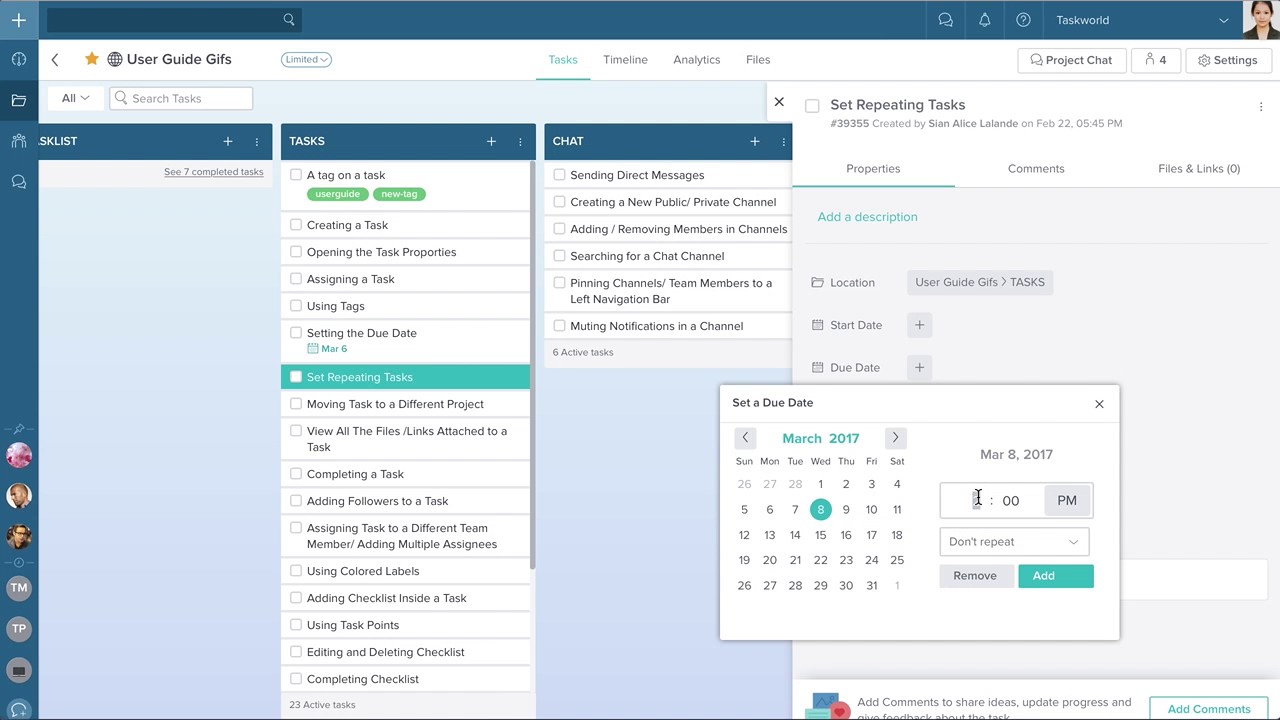The image contains a user interface (UI) screen with various elements and design components. At the top, there's a prominent blue bar with a plus sign located at the top left corner. Adjacent to this is a search bar with a reflective glass-like appearance.

Below the blue bar and search area, there's text that reads "Task World" along with several other elements. These include a droplet icon, indicating some form of status or notification. Additional icons and labels are present, such as "a meter," a folder icon, a comment bubble, and others which may not be distinctly described.

In the UI, there are sections shaded in light pink and white, possibly highlighting areas of interaction. Multiple avatar icons representing users are seen alongside the abbreviations "TM" and "TP." Below the user avatars, a task list is presented, featuring blue vector icons indicating tasks.

A series of tags are displayed under the task list, colored green and labeled with various user guide topics. These tags are categorized relevant to task management functionalities, such as "Creating a Task," "Assigning a Task," "Using Tags," "Setting the Due Date," "Setting Repeating Tasks," "Moving Tasks to a Different Project," "Viewing All Files," "Completing a Task," and more.

Additionally, capabilities like "Adding Members," "Using Code Labels," "Adding Checklists," "Completing a Checklist," "Sending Direct Messages," "Creating a New Project," "Adding and Removing Libraries," "Searching for a Chat Channel," "Pinning Channels to a Left-Hand Task Bar," and "Unifying the Channel" are mentioned, highlighting extensive task and project management features available within this UI.